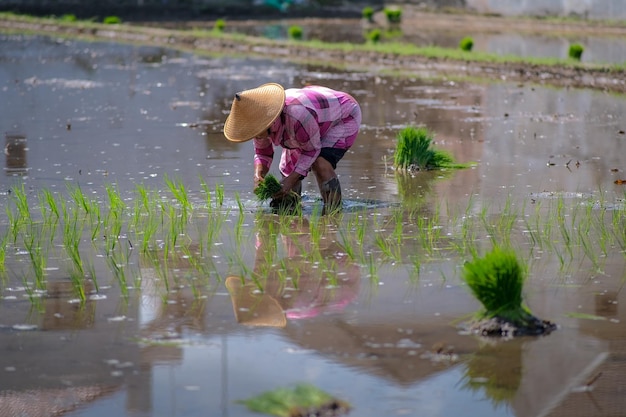This photograph captures an outdoor scene in a rice paddy, with the water reflecting a somewhat muddy, brown hue, almost like a watercolor. Centered in the image is a woman, possibly Asian, engaged in planting or harvesting young rice shoots. She is bent over, her face obscured by a traditional, pointed bamboo hat with a wide brim. The rows of vibrant green rice shoots she is concentrating on are visible, contrasting with the muddy water. The woman is dressed in a pink and white plaid shirt with long sleeves and black shorts that expose her knees and part of her shins. Though slightly shadowed, she appears to be wearing knee-high boots. In addition to the green rice shoots, there are compact tufts of plants scattered around her, some of which have been bundled together. The background reveals a green grassy edge leading to another rice paddy, and reflections of both the woman and the plants shimmer on the sunlit water, indicating it is a bright day.